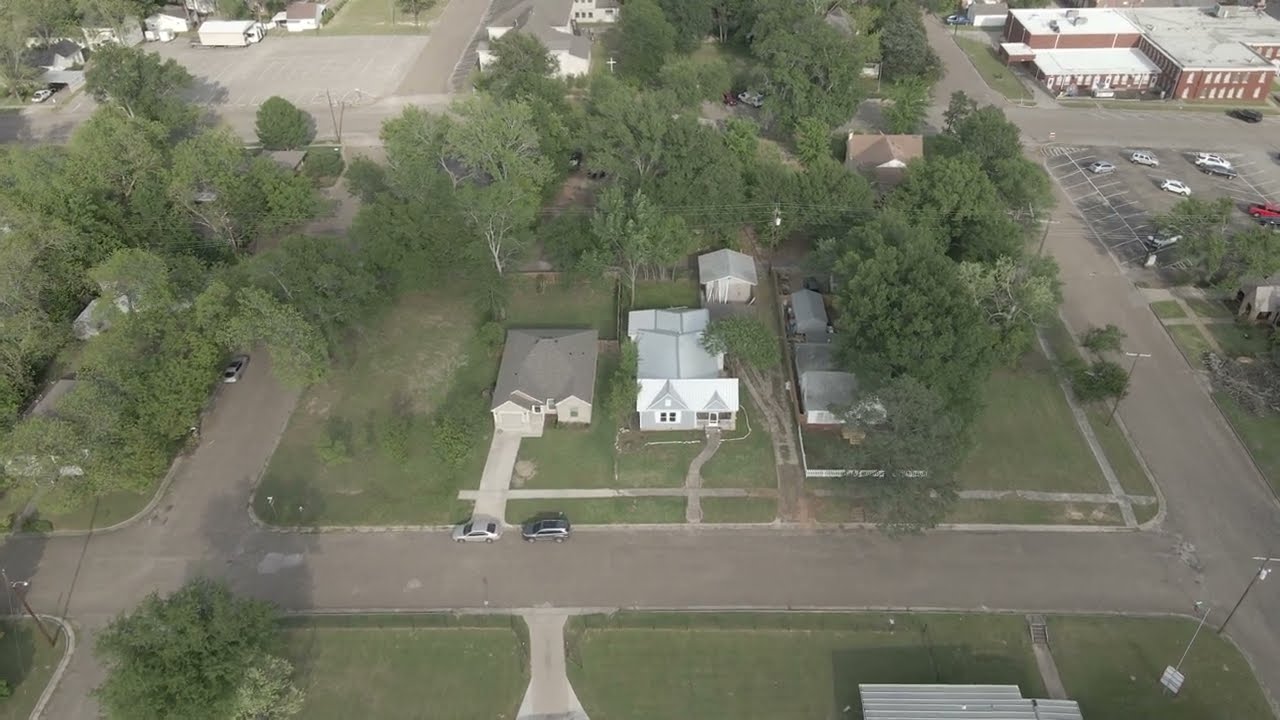This aerial photograph captures a quaint suburban neighborhood that appears to be from the mid-20th century. In the forefront, a house with a high, arched gray roof and gray front walls features a centrally placed window with a white frame. Its roof transitions to a lighter hue due to light reflection. A winding walkway leads to its entrance, slightly veering to the right before reaching the door. Adjacent on the left, another house stands with a darker gray roof and cream-colored facade, fronted by a spacious driveway and two parked cars—one silver and one darker sedan—along the light gray street.

A dense backdrop of tall, lush green trees surrounds the houses, which are accompanied by neatly trimmed green lawns. In the upper right of the image, a red brick building with a flat white roof and white-outlined windows peeks in, while in the upper left, a sizable parking lot hosts a cream and white building. The right side of the lot is filled with parked cars.

This charming, possibly historical neighborhood showcases a blend of residential and commercial areas, with various houses separated by long walkways, gates, and abundant greenery, underscoring its picturesque, serene character.